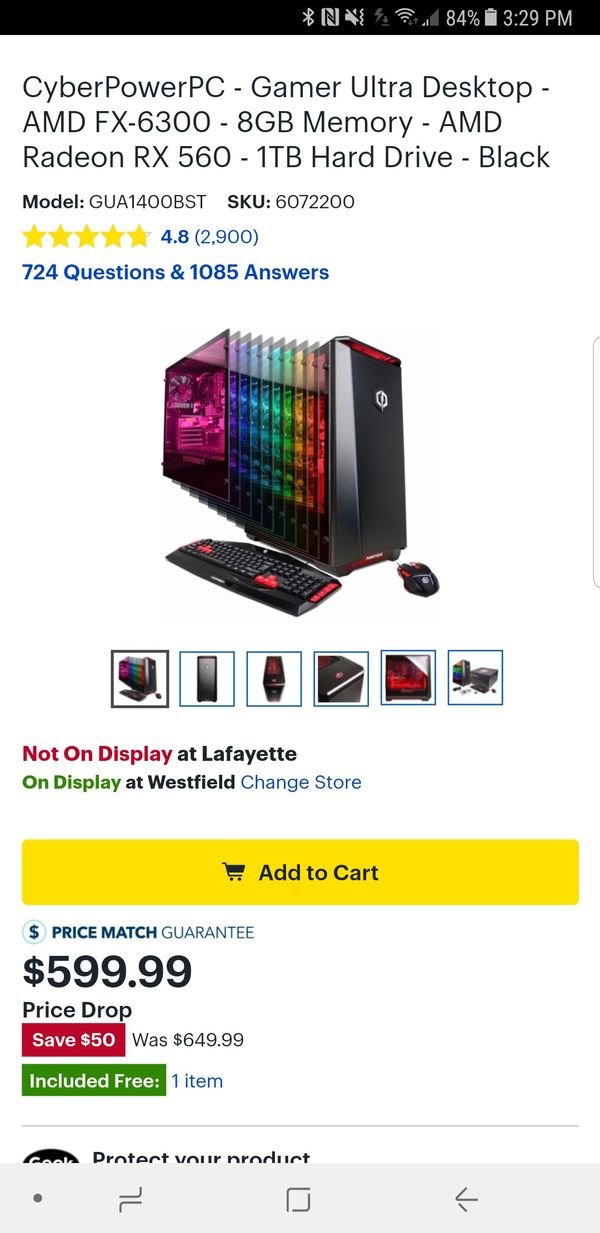This image is a screenshot taken on a cell phone, showcasing a product listing on a website. The screenshot is in portrait orientation and lacks defined borders. At the top of the image, a horizontal black bar serves as the header, displaying various phone status icons: a Bluetooth signal, network signal, silent/vibrate mode indicator, power charging lightning bolt, full Wi-Fi meter, partial network connection with one or two bars, 84% battery percentage, and a nearly full battery icon. The time shown is 3:29 PM.

Below this header, the product details are presented in black font on a white background: "CyberPowerPC GamerUltra Desktop AMD FX6300 8GB Memory and Radeon RX 650, 1TB Hard Drive, Black." The product holds a high rating of 4.8 stars based on 2,900 reviews. An image of the product is featured next, depicting a desktop computer with extending monitors displaying a rainbow of colors across different screens. Alternate images of the product are also available.

Further down, a yellow, rectangular "Add to Cart" button is prominently displayed with black text, accompanied by a price listing of $599, reduced from the original $649.